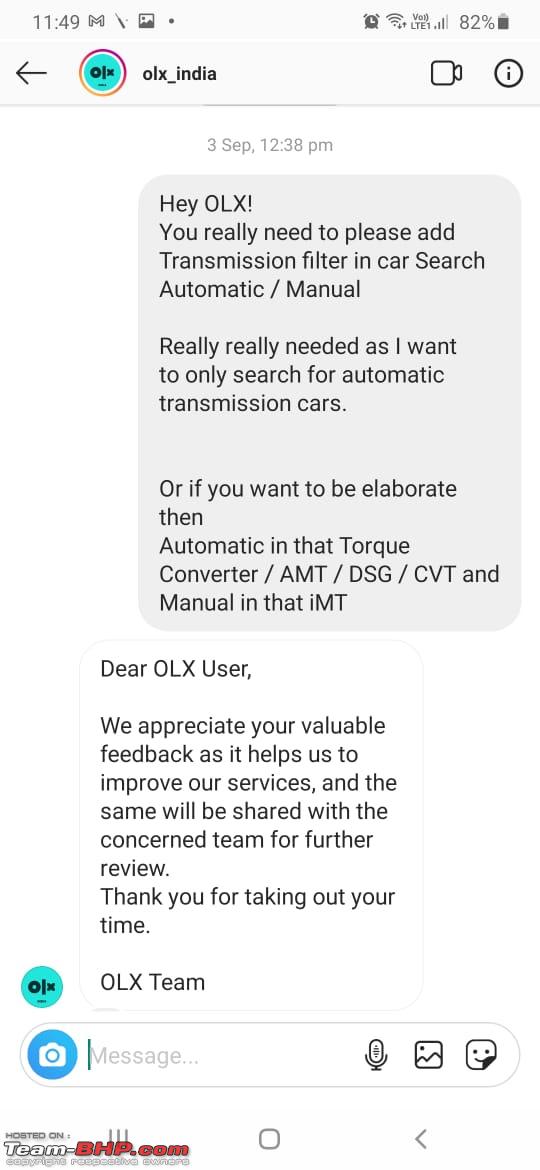Screenshot of a cell phone display at 11:49 p.m. The top bar shows a vibrant and detailed background with various status indicators: a Google Mail icon resembling a screwdriver, the Instagram logo on the far right, an active alarm icon, full Wi-Fi signal, 4G LTE connection, strong cellular signal, and a battery at 82% capacity. 

The central portion of the screenshot reveals an Instagram post by user "LOX_India," identifiable by the username at the upper left. The right side of the screen features icons including an old-fashioned video camera and a circular eye symbol. 

The core content of the screen displays a message timestamped "3 September, 12:38 p.m." on a white background with gray text. Below, a gray-background message with black text reads: "Hey OXLEY! You really need to please add 'transmission filter' in the car search/manual. It’s really, really needed as I wanted to only search for automatic car transmissions. If you want to elaborate: automatic, torque converter, AMT, DSG, CVT, and manual IMT. What the hell..."

Following this main content, a message apparently from "Jurassic user" appears, expressing appreciation for the services provided and requesting a review. The message concludes with "Thank you for your time, Oxley TV."

Below the conversation, options for sending another message, using a microphone, taking a screenshot, or adding a sticker are available. At the bottom of the screen, an overlay displays "team HBP.com," indicating the source or hosting platform.